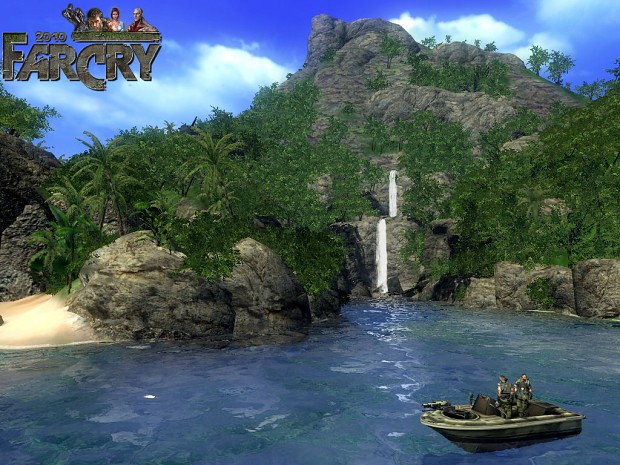This scene from the video game Far Cry captures a picturesque outdoor setting featuring a tropical lagoon with vibrant greenery and dynamic water elements. In the foreground, a camouflaged brown boat, occupied by two soldier-like figures, floats on clear blue water. This cinematic moment frames a majestic mountain at the center, adorned with lush trees and palms, and marked by two cascading white waterfalls that feed into the serene pool below. Significant large rocks and luxuriant greenery contribute to the natural splendor of this setting. The sky above is a brilliant blue, scattered with fluffy white clouds that accentuate the tropical environment. In the upper left corner, the Far Cry logo, along with the year 2010 and several characters from the game, adds an unmistakable touch of authenticity to this visually stunning snapshot. Just to the left of the mountain, a small, pristine white sand beach completes the idyllic scene.